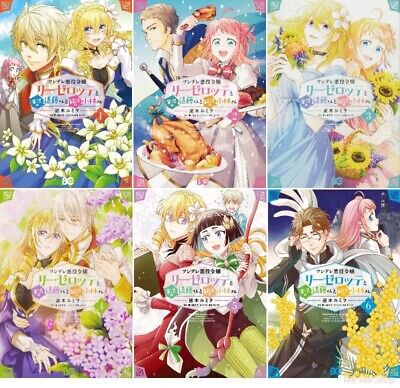The image is a poster divided into six rectangular segments, each featuring different anime-style characters, predominantly young and white, within varied thematic settings. The upper left rectangle showcases a boy and girl with gold hair, pointy chins, and large eyes, amidst flowers and a blue sky with clouds, accompanied by Chinese or Japanese labels underneath. In the upper center, a male character with brown hair and a female character with pink hair are seen, with the female carving a turkey and holding up a turkey leg. The upper right segment features two girls with golden blonde hair in blue flowy dresses, surrounded by yellow sunflowers.

On the bottom left, there's a boy with white hair and a girl with yellow hair. The bottom center shows two female characters, one with short brown hair and the other with long blonde hair, with a boy, possibly with soft tan or pinkish hair, in the background. Finally, the bottom right rectangle depicts a male character with brown hair and glasses, and a female character with pink hair. Each segment is numbered from one to six, with corresponding Japanese text labels likely identifying each segment.